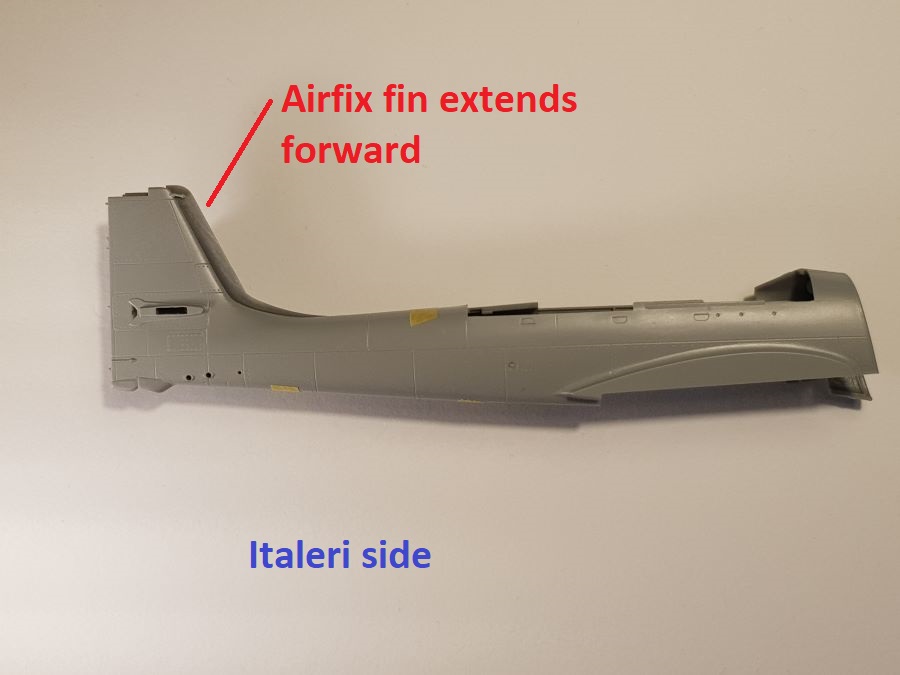The image depicts a partly assembled model airplane on a white background, resembling construction paper. The model, which is missing wings and wheels, is primarily silver or gray. A taller vertical fin is positioned towards the rear. The image contains two elements of text: in red font at the top, a label reads "Airfix fin extends forward," with a red line indicating the fin on the left side of the model. Below the airplane, in dark blue text, it reads "Italeri side," without any directional arrows. The overall presentation suggests instructional guidance, possibly for assembling the model plane. Shadows are subtly visible beneath the body of the model, adding depth to the image.